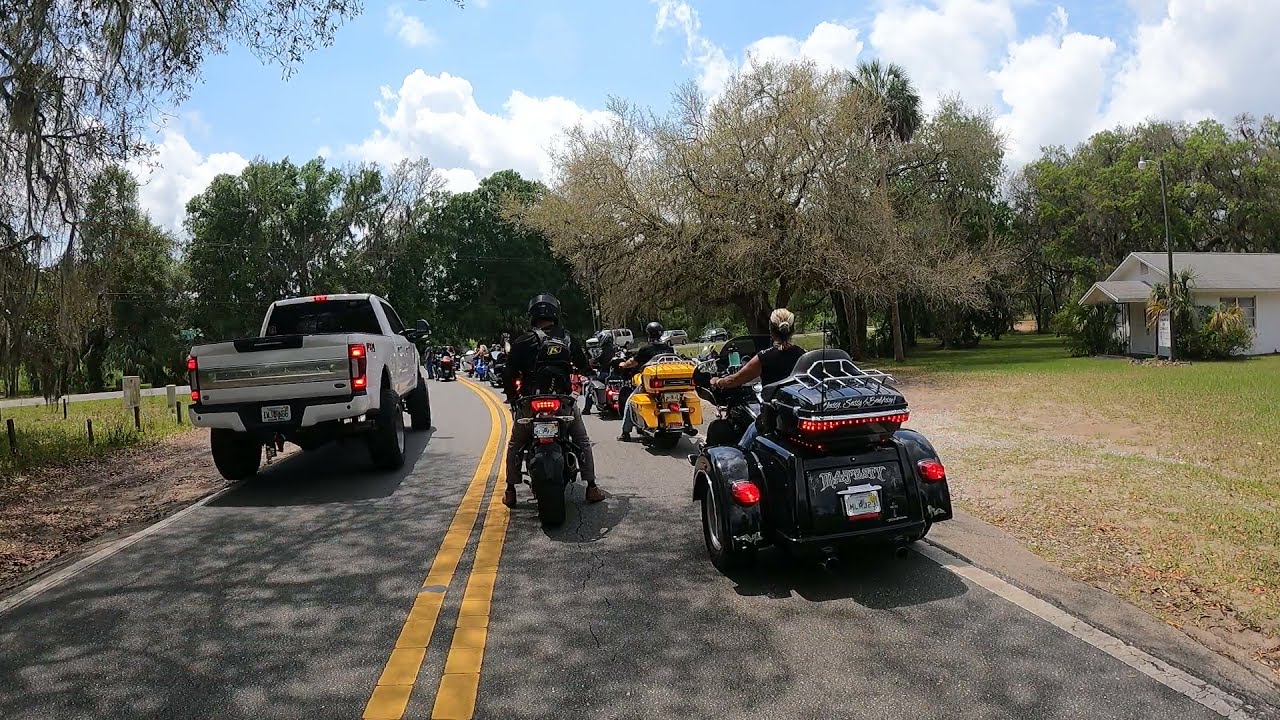The image captures a scenic outdoor setting along a small two-lane road marked by double yellow lines in the center and solid white lines on either side. Dominating the scene is a long line of motorcycles, indicative of a motorcycle gang. The lead motorcycle is a distinctive black tricycle, with a rider in black attire and a helmet. Further along, on the right side, a larger black motorcycle ridden by someone with blonde hair is visible. A yellow motorcycle and several others trail behind, although the details become sparse towards the back of the line. 

To the right of the road, there is a small white house with a gray roof, situated near a green field. On the left side, various wooden posts and stone graves contrast with the white pickup truck seen in the left lane. The background features a beautiful nature setting with trees predominantly adorned with green leaves, though some trees are bare. The sky above is a serene light blue, dotted with white clouds, enhancing the picturesque quality of the scene.